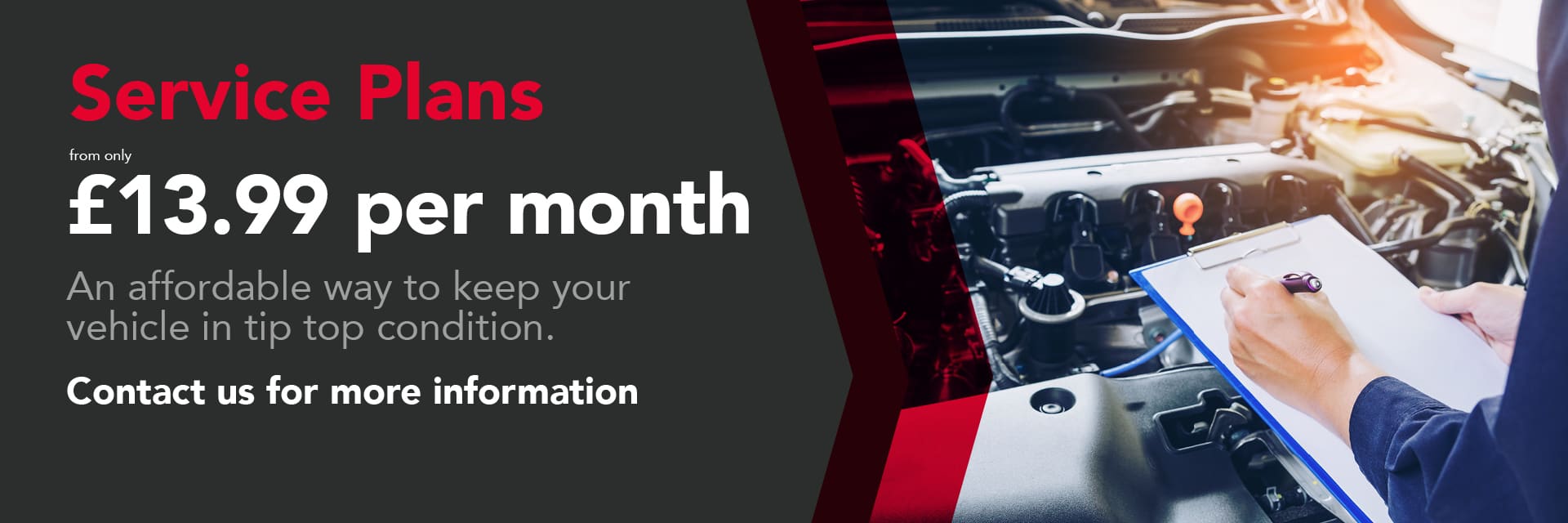The image has a 4:1 width-to-height ratio with a divided background. On the left side, a gray backdrop is present. The right side features a red diagonal separation that begins two-thirds down from the top and then reverses direction toward the bottom-left corner.

On the right side, an individual, who appears to be a mechanic, is partially visible. He is wearing a blue long-sleeve shirt and is depicted writing on a clipboard with his left hand using a black pen. The clipboard rests on his right hand. The background suggests he is inspecting a car engine, viewed from above with the hood up.

In the upper left corner of the image, "Service Plans" is prominently displayed in large, medium-red text with capitalized 'S' and 'P'. Below in smaller white text, it reads "From only". Below this, the price "13.99 per month" is shown in very large text, larger than the red text above. Further down, in light gray text of medium size, it states, "An affordable way to keep your vehicle in tip-top condition." There is a small gap, and then in similarly sized white text, the phrase "Contact us for more information" is positioned at the bottom.